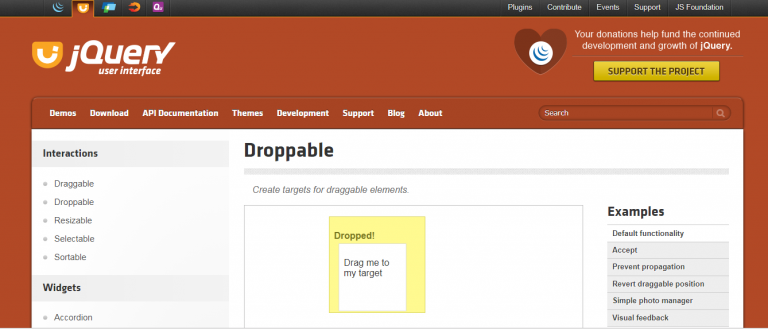A partial screenshot displays a section of the jQuery website, visible as if viewed on a laptop or monitor screen. The top section comprises a black bar with five colorful, unspecified icons on the top left, and five clickable items on the top right, one of which is labeled "Support."

The website's title, "jQuery," features a small 'j' and uppercase 'Q', accompanied by an icon depicting a smiley face within an orange half-circle. Below this, "User Interface" is textually emphasized. On the right side, a dark, shadowy heart shape encircles a motif of blue horizontal lines, reminiscent of the AT&T logo. This section encourages contributions, stating, "Your donations help fund the continued development and growth of jQuery," followed by a yellow, rectangular button labeled "Support the project," presumably leading to a donations page.

Further down, a white display area capped with a red horizontal bar lists categories in white text, including Demos, Download, API Documentation, Themes, Development Support, Blog, and About. An active search bar displays a query for "droppable," subtitled "create targets for draggable elements." A yellow square labeled "dropped" contains a smaller white square with the text, "drag me to my target," indicating interactive elements, likely part of a tutorial.

To the right, the section entitled "Examples" suggests the tutorial's context, presenting options like default functionality. Below, a gray text box details various commands such as "different lines except," "prevent propagation," "revert," "draggable," and "position," among others.

A vertical column on the left lists "Interactions," with items including Draggable, Droppable, Resizable, Selectable, and Sortable. Below this, a section titled "Widgets" shows "Accordion," while the rest of the entries remain cropped and unreadable.